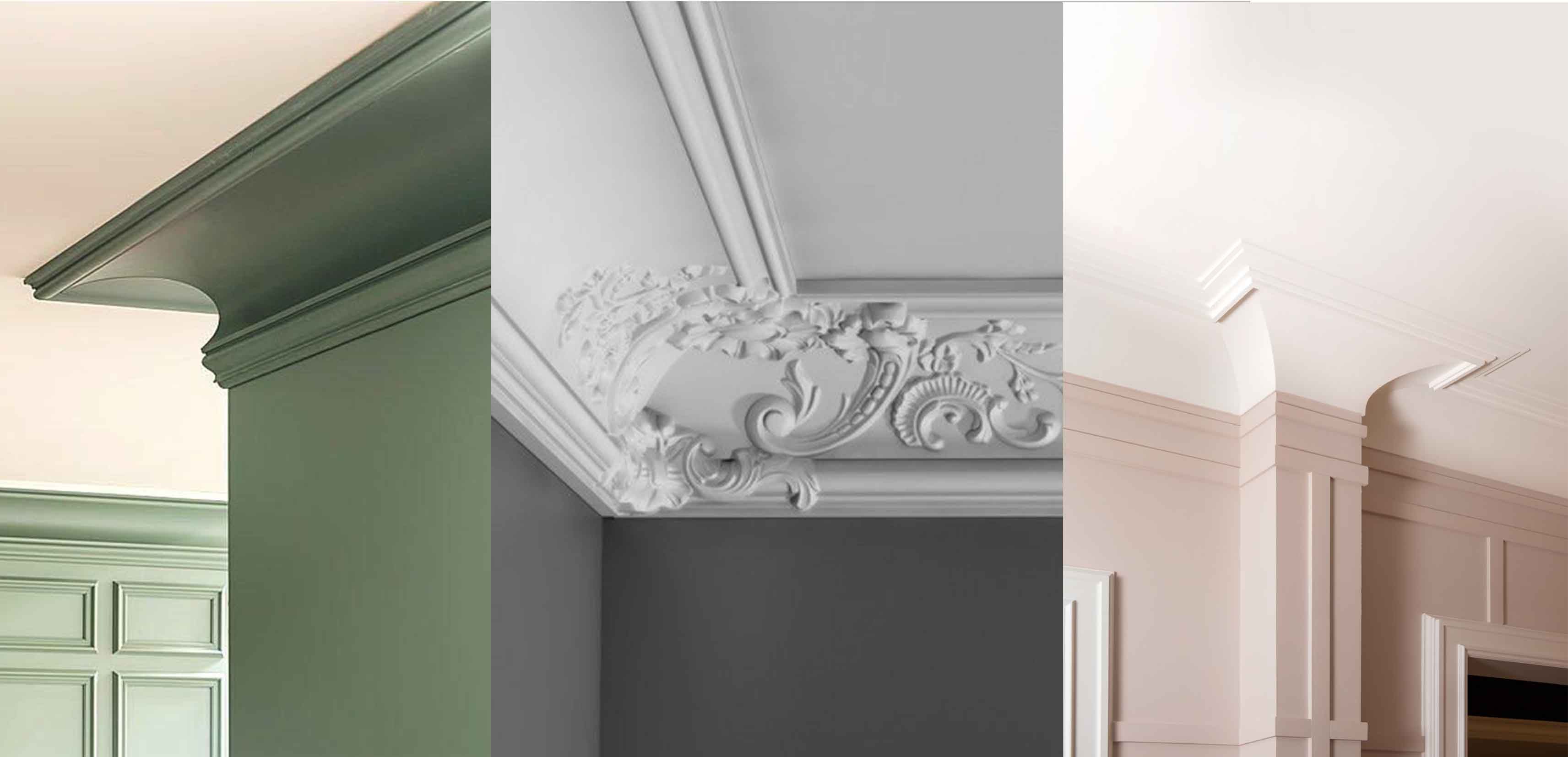The image depicts three different types of crown moldings, each showcased in a separate section. On the left, the crown molding appears modern with an olive-green wall and a subtle curve at the top, positioned against a pinkish background. The middle section reveals an ornate white crown molding featuring intricate designs of flowers, swirling patterns, and leaves against a gray wall. The right section displays a more modern crown molding against a peach-colored wall with paneling. This molding includes a column-like feature that protrudes slightly from the wall and curves into the off-white ceiling. Additionally, the bottom right corner shows the opening of a doorway.